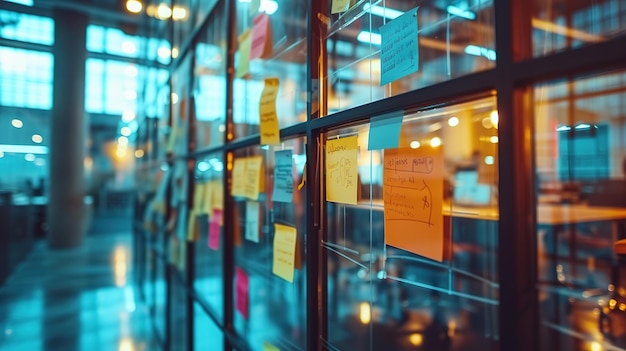In a modern office interior with a bluish-green hue, a tall white column supports the ceiling on the left, while a large, shiny black marble floor extends below. Dominating the scene is a multi-paned glass wall with a grid-like structure, framed in a brown or gold metal, dividing the visible space. Each pane of the glass wall is adorned with a variety of brightly colored sticky notes—blue, orange, yellow, and pink—all decorated with illegible handwritten messages. The background reveals a conference table surrounded by chairs and illuminated by reflective lighting, adding to the modern glow of the setting. Through the clear glass and beyond the sticky notes, a hallway and additional interior structures hint at a restaurant or store atmosphere, enhancing the image's dynamic and contemporary feel.